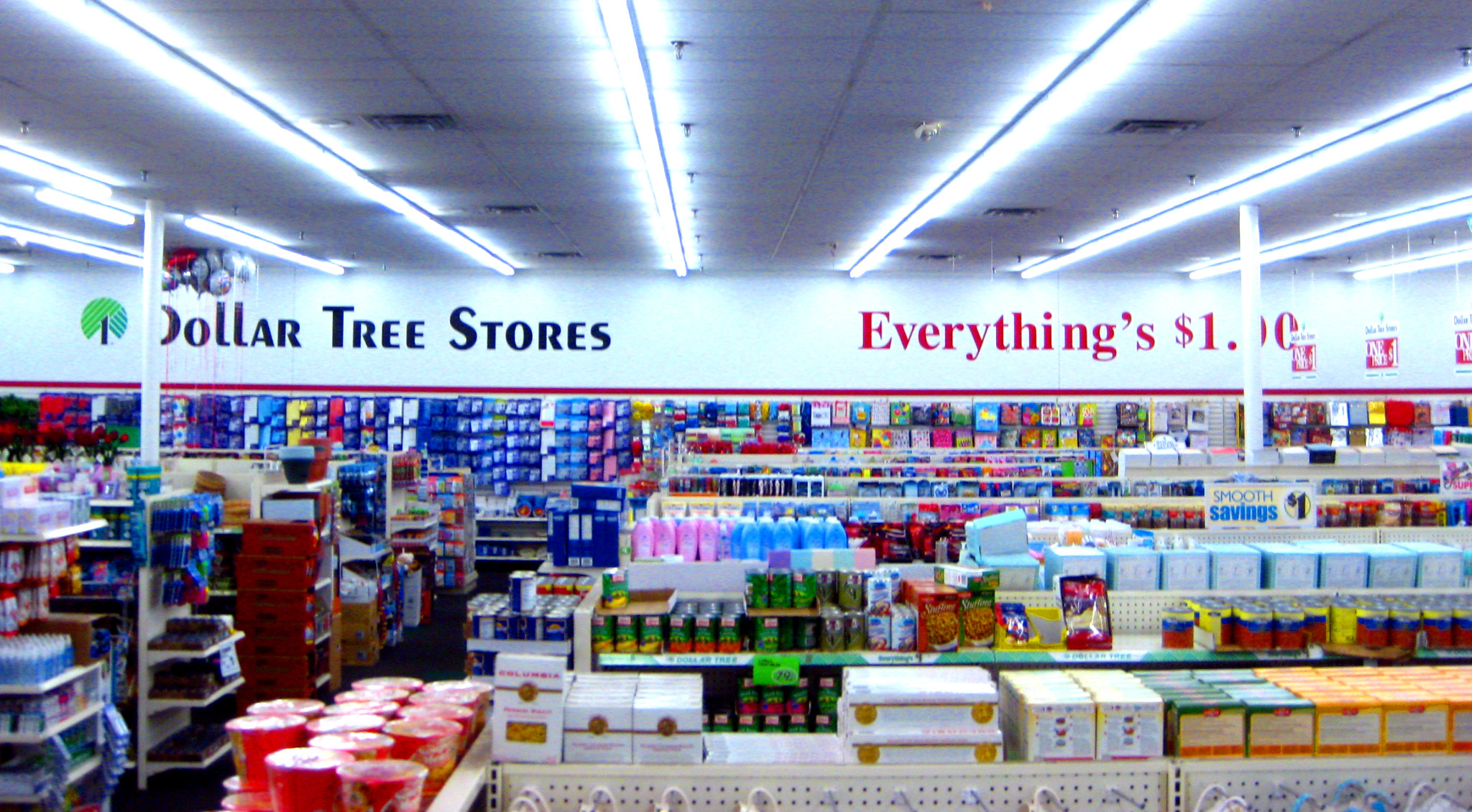This image captures the bustling interior of a Dollar Tree store. The ceiling at the top of the frame is lined with fluorescent lights that illuminate the aisles below, extending towards the back of the store. Dominating the background is a wall adorned with bold black text that reads "Dollar Tree Stores," accompanied by the store's recognizable green logo to the left. To the right, in striking red font, the sign declares, "Everything's One Dollar." 

In the foreground, numerous well-organized shelves are brimming with a variety of items. Visible on these shelves are beverages, cups, snacks, and possibly boxes of tea, showcasing the wide range of products available for purchase. Along the back wall, a neatly arranged display features a multitude of gift cards, each securely attached and ready for shoppers to peruse. The image effectively conveys the essence of the store, highlighting its promise of affordability and diverse inventory.